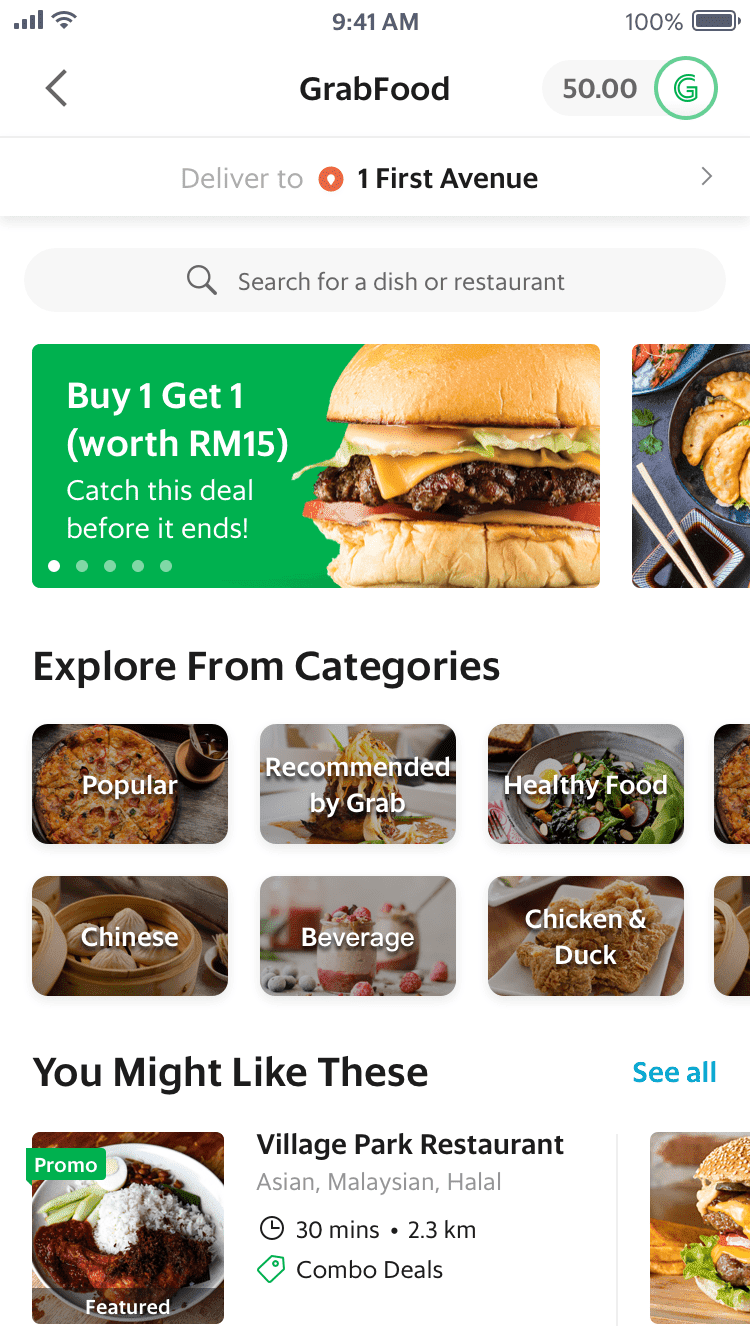A screenshot of a food delivery app displayed on a smartphone screen. The background is predominantly white. Across the top left, there are signal bar and Wi-Fi icons, both indicating full strength. Centered at the top, the time reads "9:41 a.m." To the top right, the battery status shows "100%" with a fully shaded charging icon.

Below the status bar, the name of the app, "GrabFood," is boldly centered. To the left of "GrabFood" is a left-pointing arrow, and to the right, it reads "50.00," next to a green outlined circle with a capital letter "G," likely representing GrabFood's credits or currency.

Underneath, there’s a delivery address bar displaying "Deliver to 1 First Avenue," followed by a search bar with a magnifying glass icon and placeholder text, "Search for a dish or restaurant."

The main section features promotional content. The first ad, taking up about one-fifth of the screen, showcases a close-up of a cheeseburger with toasted buns, cheese, a burger patty, a tomato slice, and lettuce or pickles. Against a green background, the text reads "Buy One Get One (worth RM 15). Catch this deal before it ends!" A sliver of a secondary ad featuring a wok with gyoza and chopsticks is partially visible, suggesting more deals available by swiping right.

Following the promo section, the app offers an "Explore from categories" section with two rows of horizontal rectangle categories. Each category has a photographic background with white text. Categories include:
- Popular (pizza background)
- Recommended by Grab (fancy plated dish)
- Healthy Food (salad/veggies)
- Chinese (bamboo steamer with baozi)
- Beverage (fancy or iced lattes)
- Chicken and Duck (fried chicken)

At the bottom third of the screen, under the title "You might like these," there's a blue "See All" button to the right. A featured listing for "Village Park Restaurant" including labels like "Asian," "Malaysian," and "Halal," promises combo deals. The listing notes a 30-minute delivery time or 2.3 kilometers distance, with a promo image of a meat and rice dish.